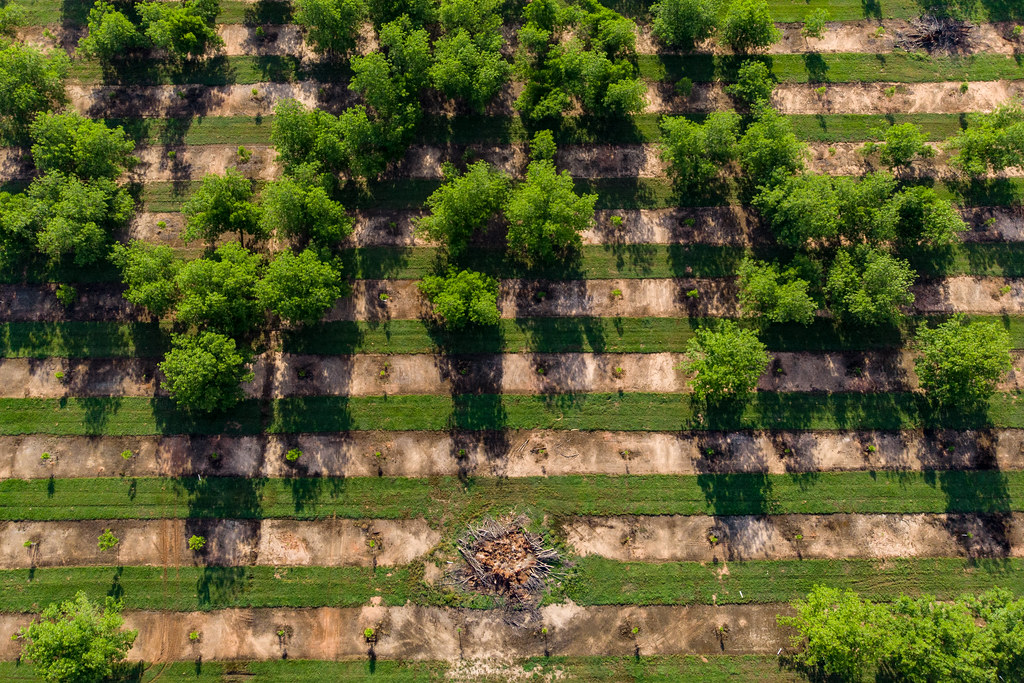This is a detailed overhead color photo of a tree farm displaying a meticulously organized landscape. The farm features alternating, evenly spaced rows of dirt and green grass that create a striped pattern stretching from the top to the bottom of the image. In the dirt rows, trees are planted in orderly, interspersed spaces. The bottom half of the picture is primarily filled with young, recently planted trees, while the upper half showcases more mature, fully-grown trees. Toward the center of the bottom third of the image, there is what appears to be a burn pile comprised of twigs. The entire scene is devoid of people, presenting a tranquil and methodically cultivated agricultural landscape.